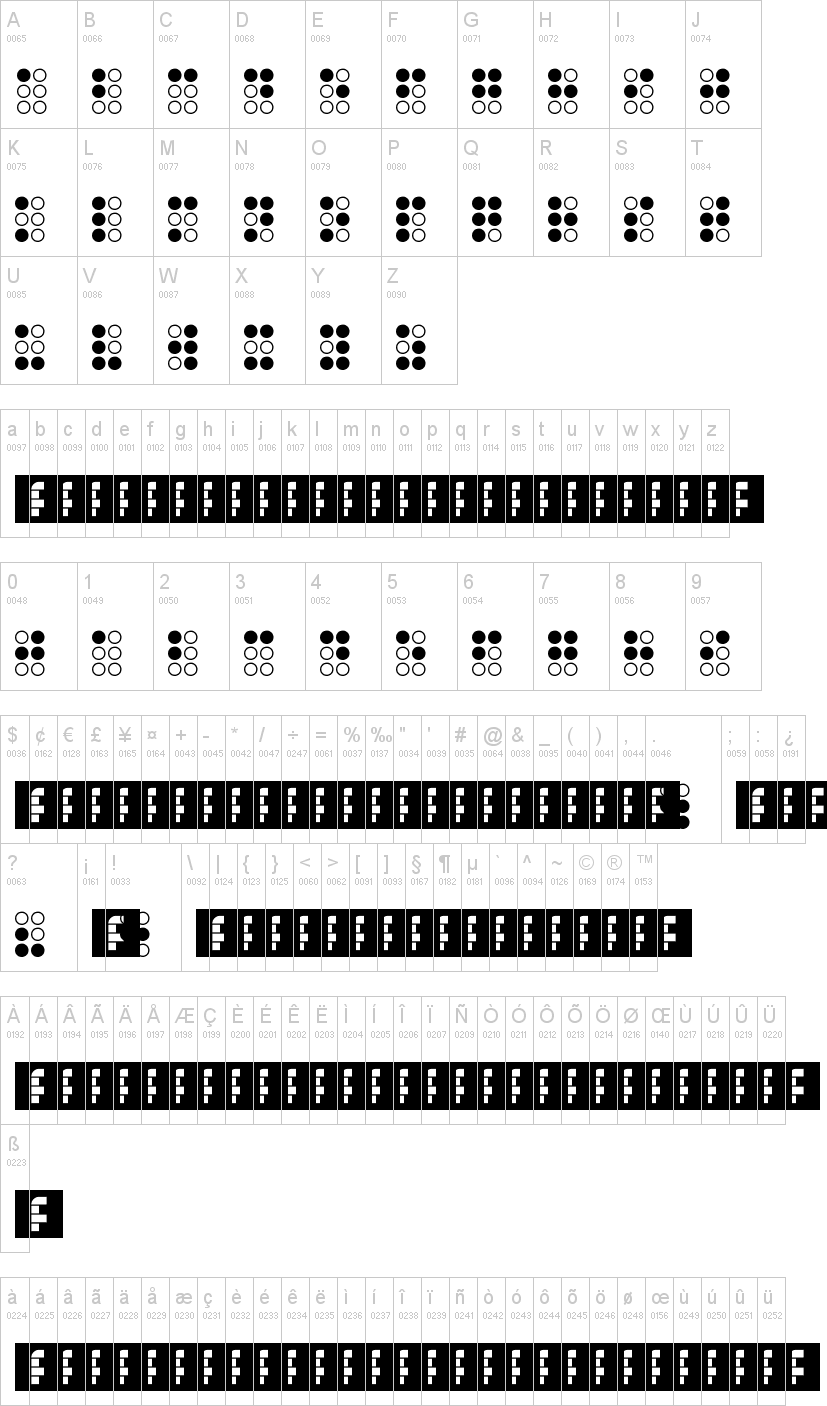This black-and-white chart showcases a comprehensive array of characters and symbols. The top section features a sequence of letters from A to Z, each contained within boxes housing six small circles. The circles are arranged in a consistent pattern, but their color schemes vary—some are black, others are white. For instance, in the first box for the letter A, the top-left circle is circled in black.

Beneath the alphabet sequence, the chart extends to include numbers 0 through 9, each again accompanied by six differently arranged circles. Special characters from a standard keyboard, along with their unique circle patterns, follow next. The subsequent rows present various letters, particularly vowels such as A, E, I, O, and U, in several formats including both uppercase and lowercase versions.

Additionally, there are characters that seem to be variants or special types, like perhaps a German "ß". Each character comes with an assortment of intricate markings or symbols displayed below them, adding another layer of detail.

The chart is meticulously organized and monochrome, eschewing any color to maintain a clean, visually consistent design.